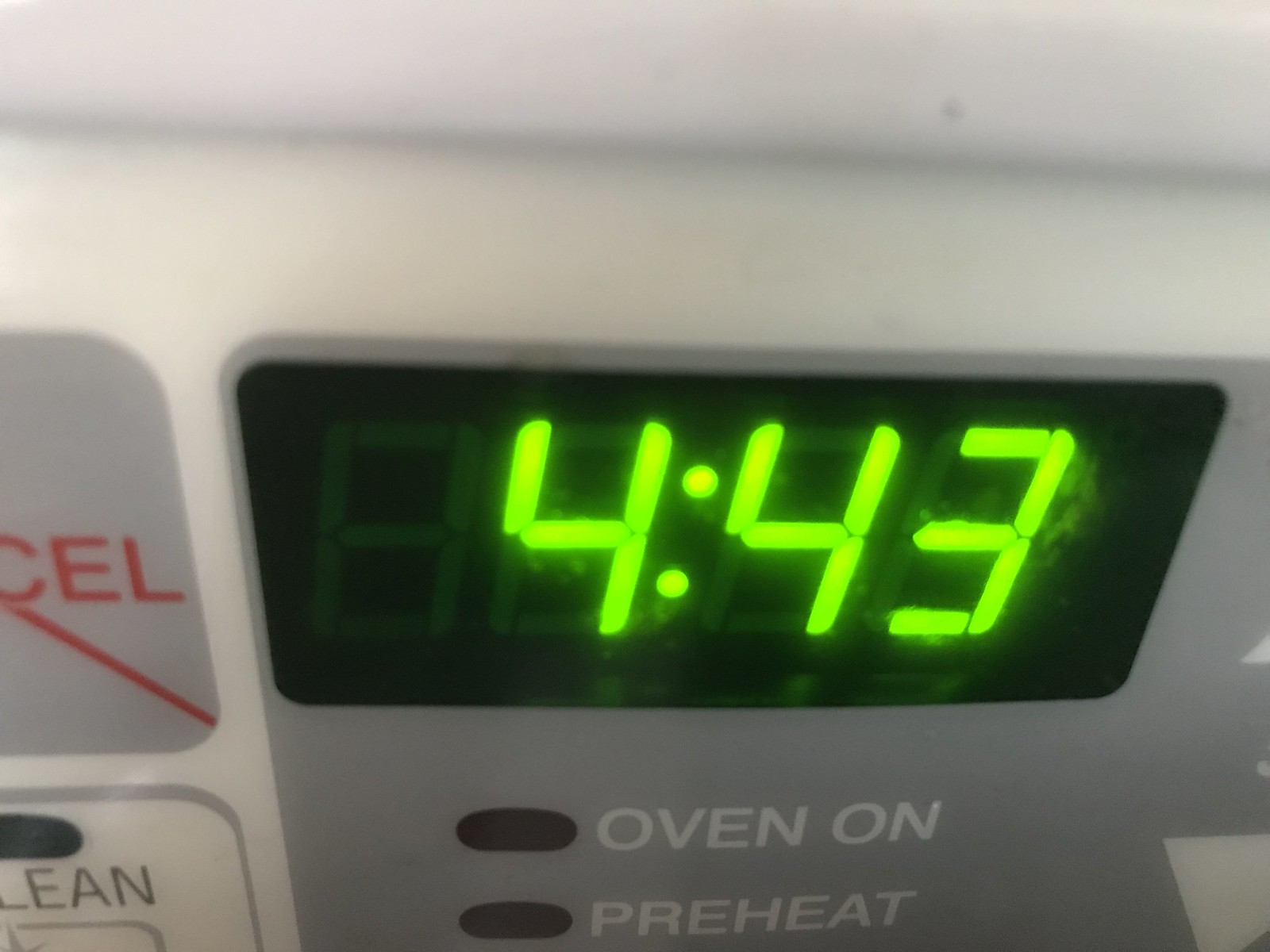This close-up color photograph captures a detailed view of the top right-hand corner of a white kitchen oven, possibly a microwave or toaster oven. At the center, a black digital display showcases glowing green digits reading "4:43," likely indicating the current time. Below the display, white text set against a gray background reads "oven on" and "preheat," with small black dots to the left of each phrase. To the left of the display, partial view of control buttons includes one gray button labeled "CEL" with red detailing, suggesting a "cancel" function, and another white button with gray letters that spell "LEAN," likely part of the word "clean." The surrounding area of the panel is a combination of white and gray tones.